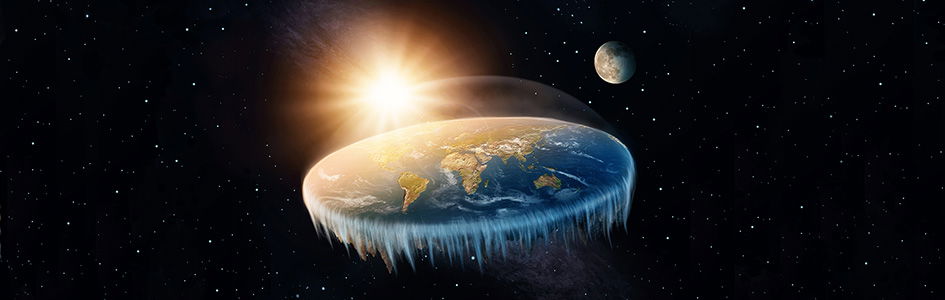The illustration portrays a cosmic scene with a black background speckled with stars. Positioned at the center is a flat representation of Earth, resembling a disk with ocean waters appearing to flow off its edges like icicles. This flat Earth's surface features recognizable continents such as South America, Australia, Asia, and Africa, rendered in typical globe colors with greenish landmasses and blue oceans. Surrounding the flat Earth, a glowing object—presumably the Sun—casts bright rays from above, partially obscuring the details on the disk with its intense light. To the right of the scene, the Moon is visible, half shrouded in darkness, enhancing the celestial ambiance of the entire illustration.